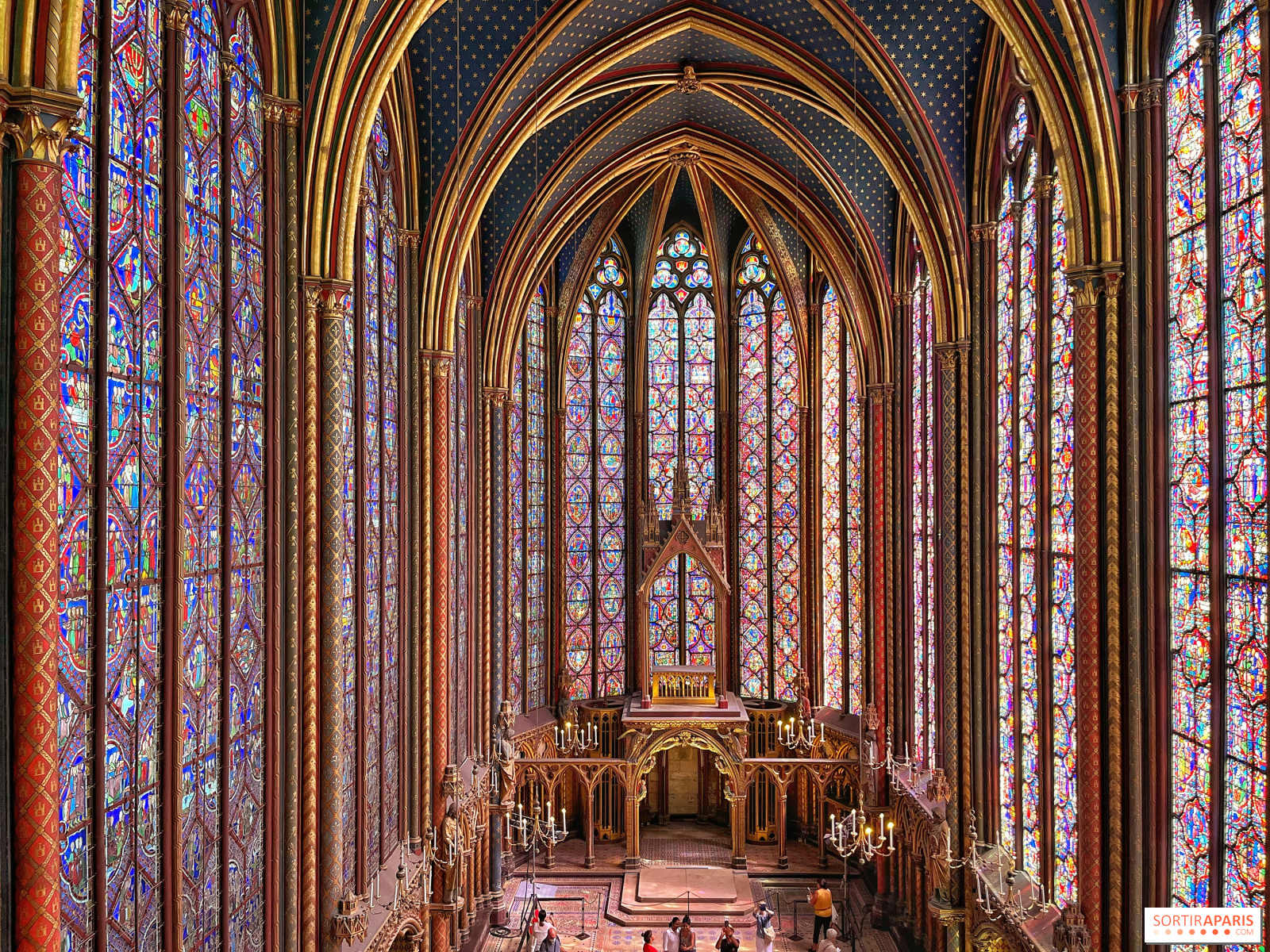The image depicts the grandiose interior of a Gothic-style cathedral, showcasing its architectural magnificence. The scene is enveloped by towering arched beams and adorned with stained glass windows on every wall, these windows framed with gold trim and casting vibrant colors throughout the space. The ceiling soars above, featuring an intricate grey and white peppered texture interspersed with blue and gold polka dots. Embossed wood finishes, possibly overlaid with metal, add to the opulence of the cathedral's structure. Dangling from the ceiling are numerous elegant chandeliers, their light illuminating the golden floor below, where groups of people meander, likely visitors. Intricately carved figures and statues line the sides, along with long, substantial ropes reaching from the chandeliers to the lofty ceiling. The image centers on a series of steps leading up to what appears to be the altar area, flanked by impressive candelabras, although the actual altar is not visible, hinting at a deeper area possibly housing the altar and an organ.